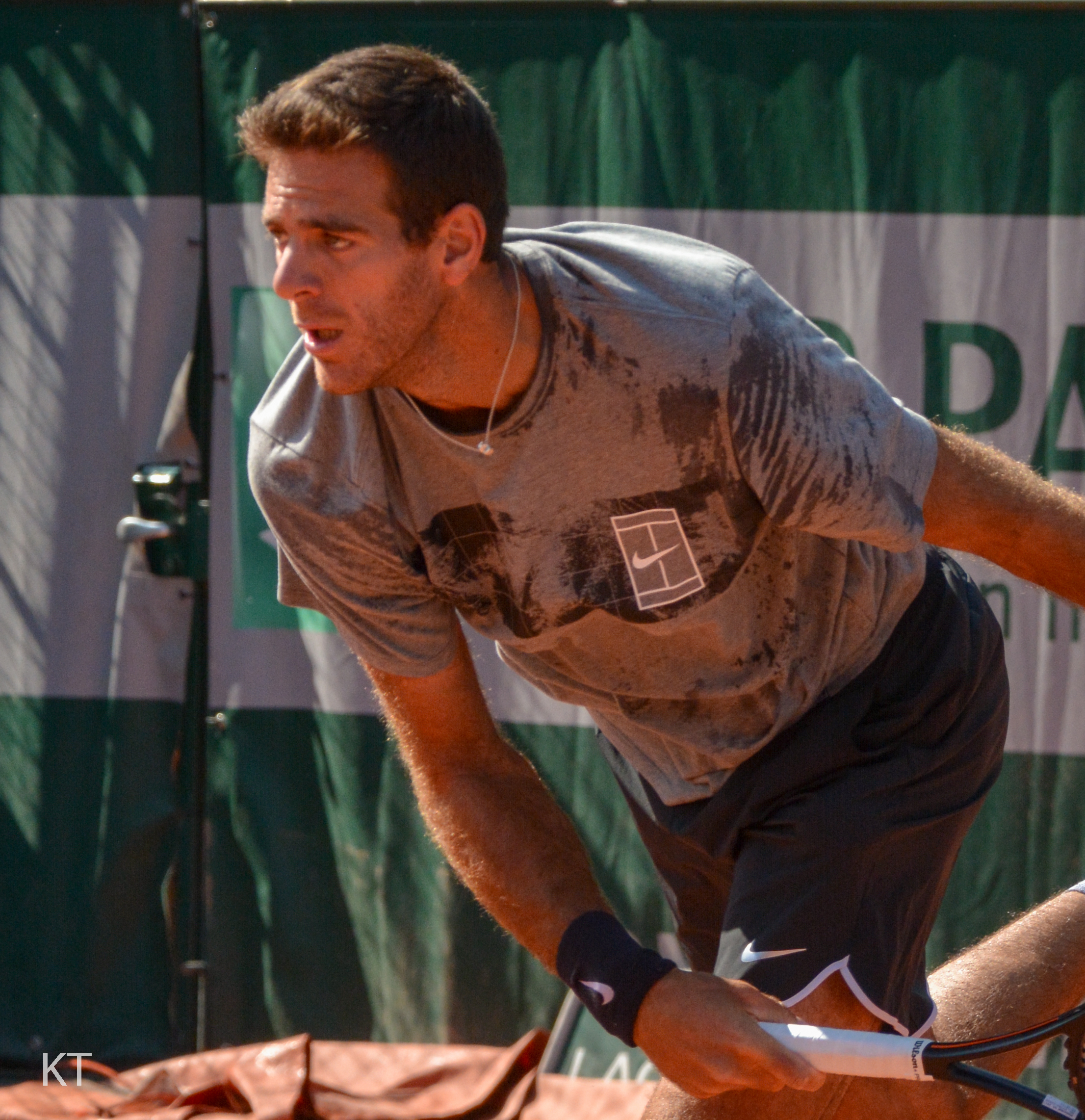This image captures a moment from an outdoor tennis match, featuring a male tennis player in the midst of action. Positioned on the right side of the frame, he is dressed in a gray Nike shirt, black Nike shorts, and Nike wristbands on both wrists. In his right hand, he holds a black and white tennis racket, which appears to be lowered around his knee, suggesting he has just completed a serve. The player has one leg up, as if he is either running or stepping forward, and his body is slightly hunched indicating an intense focus on the game.

The player has short, spiky brown hair, and a small silver necklace that may feature a ring. His facial features include a bit of stubble, and his sweat-soaked shirt indicates the warm climate of the setting. Behind him, a green tarp with white lines and some green lettering partially obscures an indistinguishable logo or insignia. Additionally, a hint of an orange tarp is visible at the bottom of the screen, creating a contrasting backdrop. In the bottom left corner, white superimposed writing reads "KT."